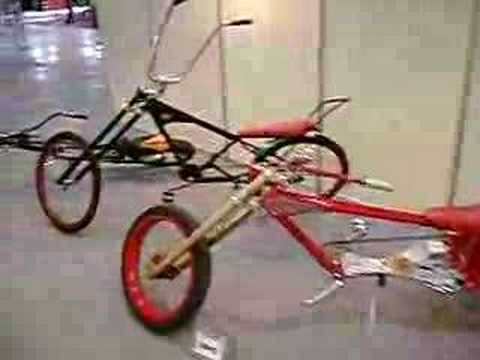The image appears to be a heavily compressed, low-resolution screenshot from an indoor video, exhibiting significant macro blocking. The setting includes tan walls and a shiny floor, which might be carpet. At the center are three bicycles, featuring long frames that distinguish them from typical bikes. 

The closest bike, positioned on the right and oriented east, has a red metal frame with silver and gold handlebars, and a black wheel with a red hub or inner rim. Just behind it, slightly to the left, is a black bicycle with a pink seat and tall handlebars that require an upright riding position. This bike also likely has a black wheel with a red center. The third bicycle, also black, lies on its side to the left of the other two. All three bicycles have long frames, indicative of a specialized design. Due to the image’s poor quality, finer details are difficult to discern.